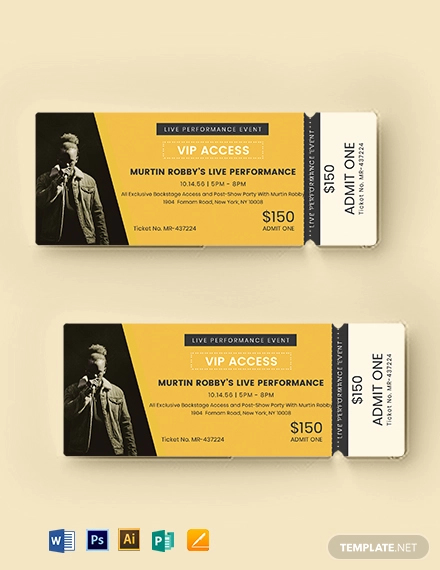This image showcases two concert tickets for Merton Robbie's upcoming live performance, against a pink background. Each ticket is long and rectangular, with one slightly overlapping the other, positioned so that the top ticket is slightly to the left. The tickets have a striking design, divided into three sections from left to right.

The left section features a black background with a shadowed photograph of a person, presumably Merton Robbie, singing into a microphone. Centrally aligned in a minimalistic white font is the text "VIP ACCESS," enclosed within a thin white border.

Moving to the middle section of the ticket, a diagonal divide transitions from black to gold, listing essential event details in white lettering, including the date "10-14" and the time "5 p.m. to 8 p.m." Below, it reads "Merton Robbie's Live Performance," accompanied by the ticket price "$150" and the phrase "Admit 1." The ticket number appears here, though indistinctly, potentially reading "477224."

The rightmost section contains the ticket stub, predominantly white with a black border separating it from the main ticket. Oriented sideways, details here reiterate the "$150" price and "Admit 1" phrase. The corner of the stub subtly displays "template.net." Additionally, symbols for "PS," "AI," and "PowerPoint," along with a yellow box and a red pin, suggest the image might be a digital template.

In summary, the detailed design of these VIP access tickets for Merton Robbie’s concert captivates with its black, gold, and white color scheme, and a notable photograph, promising an exclusive live performance experience.